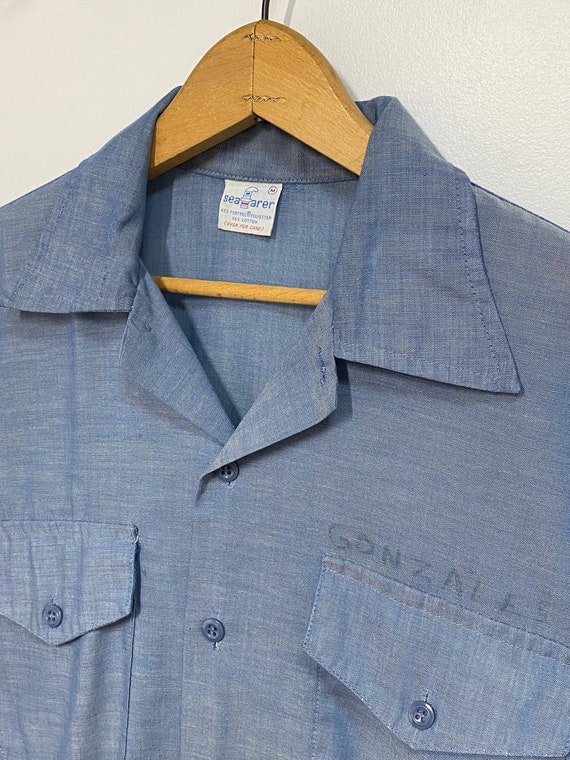This image depicts a neatly pressed, light blue button-down work shirt hanging on a light wooden hanger with a partially visible metal hook, set against a clean white background. The shirt features a collared design, with all buttons fastened up the front and both chest pockets securely buttoned shut. The right-side pocket bears the name "Gonzales," although the text appears somewhat faded, indicating frequent use. The shirt is in good condition, relatively clean, and free of missing buttons. Additionally, the tag on the shirt reads "CR," identifying the manufacturer. Overall, the shirt presents a professional yet worn appearance.